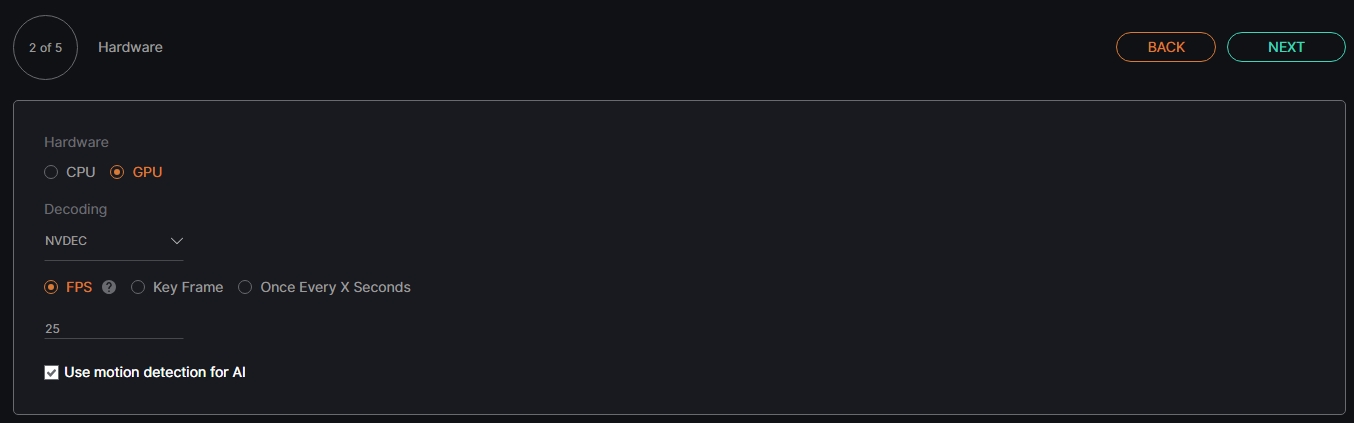This screenshot covers the full width of the screen but has a relatively small height, set against a jet-black background. In the upper left corner, a small gray circle indicates "2 of 5" and the word "Hardware" next to it. The center of the image is mostly empty, creating a stark contrast with the detailed elements on the far right.

On the right side of the screenshot, two buttons are noticeable. The first button is outlined in red and labeled "Back" in red lettering. Adjacent to this, a slightly larger button is outlined in light blue with the label "Next," also in light blue.

Below these buttons, there is a rectangular box with a light gray trim. At the top of this box, the text "Hardware" is displayed, with two options underneath: "CPU" and "GPU." Further down inside the box, under a section titled "Decoding," the option "VBS" has been selected from a dropdown menu.

At the bottom of the image, in white text, there is an option labeled "Use motion direction for AI," which has been clicked on, as indicated by a checkmark.